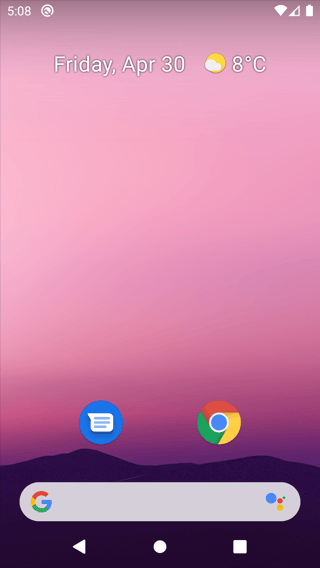A detailed screenshot of a smartphone background captures various on-screen elements against a gradient backdrop. In the top left corner, the time "5:08" is displayed in light gray, accompanied by a "No Signal" icon—a circle with a slash through it. Further to the right, the status bar includes a Wi-Fi icon, followed by signal bars showing two or three bars, and finally, to the far right, a fully charged battery icon. 

The background transitions from a dark purple at the top to a lighter purple in the middle, and back to a darker purple at the bottom, forming shapes reminiscent of mountain peaks in deep purple. Centrally positioned at the top, "Friday APR 30" is shown in white text, along with an icon displaying a sun behind a cloud, next to the temperature of 8 degrees Celsius.

In the lower section of the screenshot, various icons and elements are arranged. To the left-middle, there is a messaging app icon resembling a speech bubble. To its right is the Google Chrome app icon. Below, a Google search bar is present. The bottom row features navigation icons: a left-facing arrow on the left, a white circle in the center, and a white square on the right.